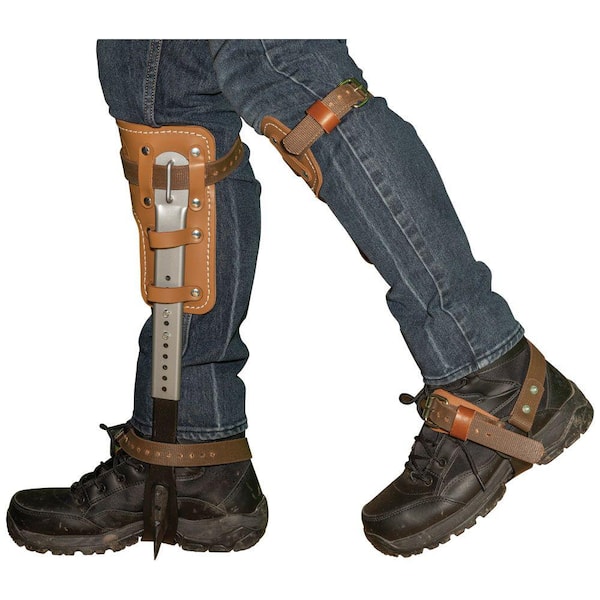This image showcases the lower legs of a person wearing blue jeans and black shoes against a white background. The jeans feature a faded seam, transitioning into lighter shades of blue. The left leg, closer to the right side of the photo, is adorned with a leather knee strap sitting just below the knee, while the right leg displays a more complex setup. Affixed beneath the knee of the right leg is a brown leather and metal brace used for added support, potentially for mountain climbing or relieving shin pressure. This brace includes a silver and black bar extending down to the shoe, terminating in a black section with spikes. Leather straps also encircle the foot, adding to the structured setup. The overall scene has a functional, possibly product-focused aesthetic, in line with a shopping listing style photo.